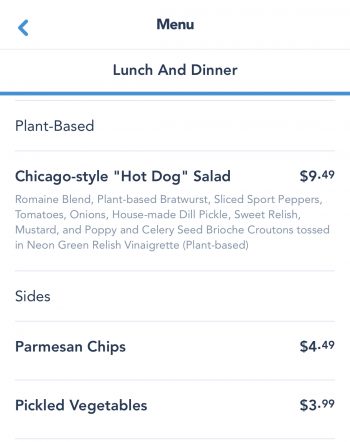This image is a screenshot from either a mobile device or a tablet, displaying a plant-based section of a menu from a website or app. The layout features a white background with black text, some bolded and in varying sizes for emphasis. In the top left corner, there is a blue back arrow indicating the option to return to the previous screen.

The main focus is a lunch and dinner menu, highlighted by a blue underline beneath the "Lunch and Dinner" header. This section is specifically dedicated to plant-based options. The first item listed is a "Chicago Style 'Hot Dog' Salad" priced at $9.49. The detailed description of the salad mentions a romaine blend with plant-based bratwurst, sliced sport peppers, tomatoes, onions, house-made dill pickles, sweet relish, mustard, and croutons made from poppy and celery seed brioche. This salad is tossed in neon green relish vinaigrette and labeled as plant-based.

Additionally, the screenshot includes a section for sides, although it is not fully expanded. The available sides listed are Parmesan Chips for $4.49 and Pickled Vegetables for $3.99.

Overall, the screenshot provides a glimpse of a plant-based menu selection, including a detailed description of a unique salad option and brief mentions of available sides.